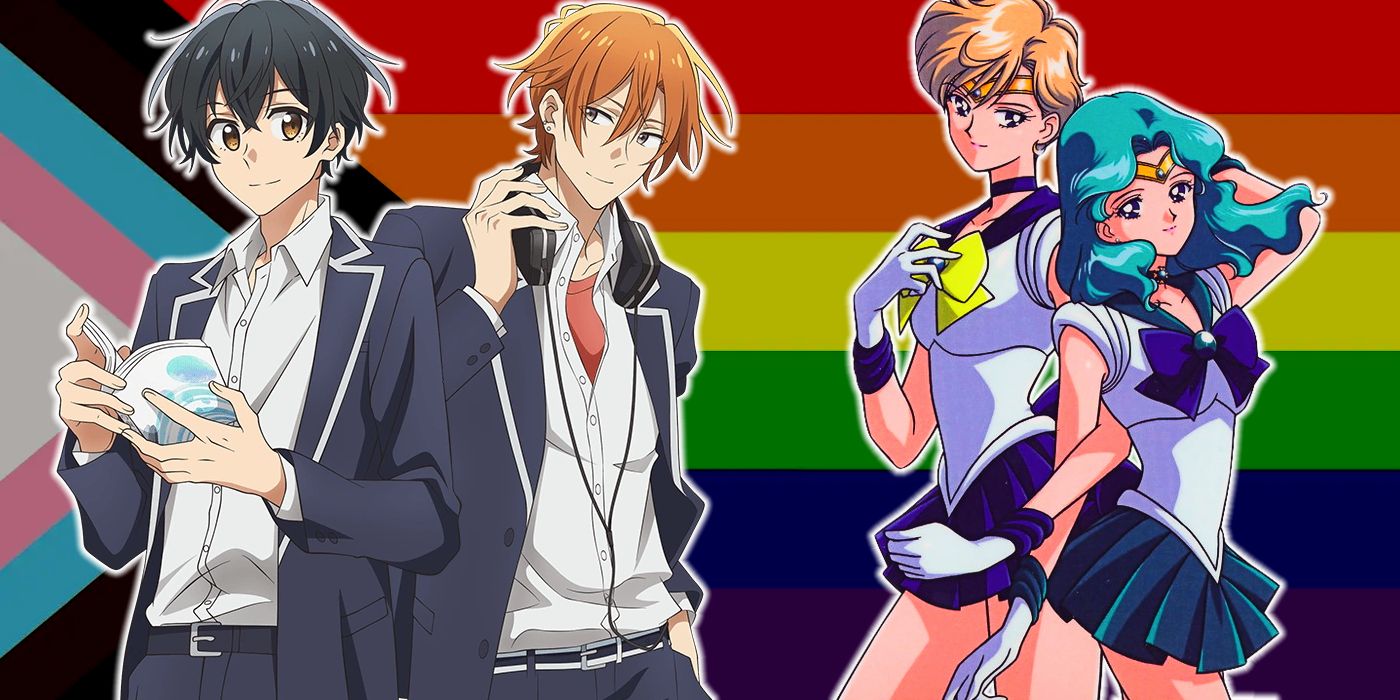The image is an animated depiction of four anime characters set against a background of six rainbow-colored stripes—red, orange, yellow, green, blue, and purple—with additional white, pink, blue, and black stripes extending inward from the left. On the left side of the image are two male characters, both wearing dark blue tux jackets and white button-up shirts. The first male, who has black hair and brown eyes, is holding or reading a book. The second male has light brown, almost orange-colored, hair and is wearing headphones around his neck, with an orange undershirt visible beneath his attire. On the right side are two female characters dressed in tight-fitting white tops with short skirts; one skirt is blue, and the other is teal. The first girl has blue hair, while the second has light brown, nearly blonde hair, and they both appear to be posing for a photo.